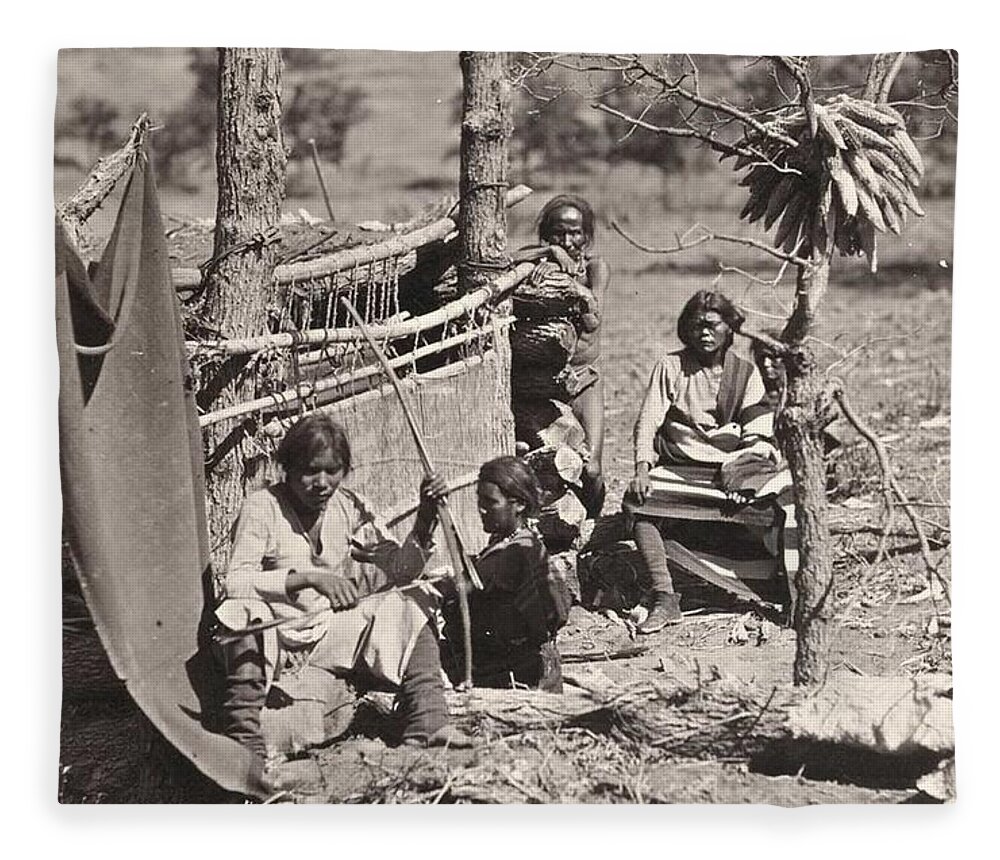This black-and-white photograph captures five indigenous individuals in a remote, wooded area, likely an exotic locale such as New Guinea. The people, dressed in very simple clothing, are gathered outside a rudimentary, man-made shelter constructed from sticks, branches, and tarps. The shelter is securely tied with rope and features a cloth door and rooftop. Three of the individuals are seated—one on a log, another on the ground, and a third on a possible stool—while a fourth person stands leaning against the hut and a fifth person is partially obscured in the background, possibly a woman. The individuals, with long hair and darkened skin, are surrounded by small trees, dried grasses, and dirt. One person prominently holds a bow and arrow. At the top of one tree, a bunch of drying corn cobs is visible. The photo, taken in shades of black, white, and gray, appears to be from a time and place not well-civilized, emphasizing the secluded and raw setting of the scene.